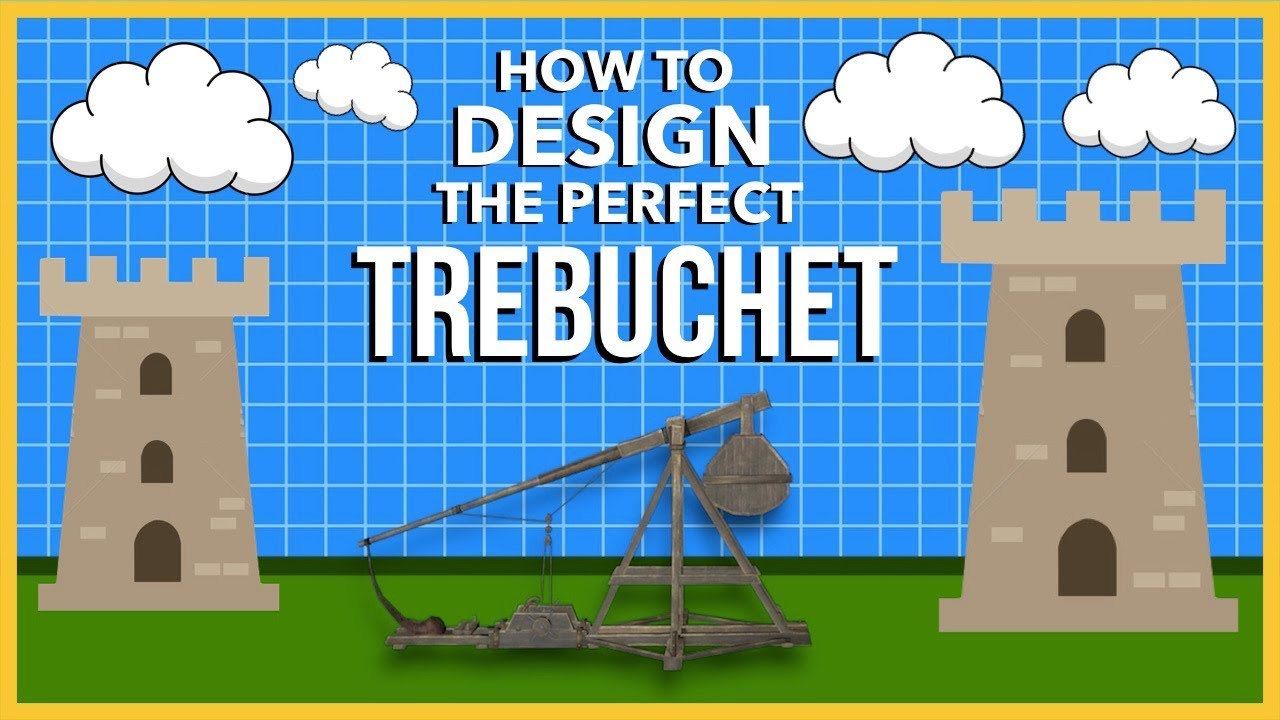The image is an illustration themed around trebuchets, designed either as a YouTube thumbnail or a presentation slide. It prominently features the title "How to Design the Perfect Trebuchet" in white text with a strong black shadow at the center. The backdrop is a blue architectural grid, resembling graph paper, accentuated with white lines. In the upper portion, there are four cartoon-like white clouds, while on the left and right sides stand illustrated medieval towers of varying sizes. A realistic trebuchet aiming to the right is centered at the bottom, situated above a strip of green field. The entire image is neatly framed with a thin yellow border.